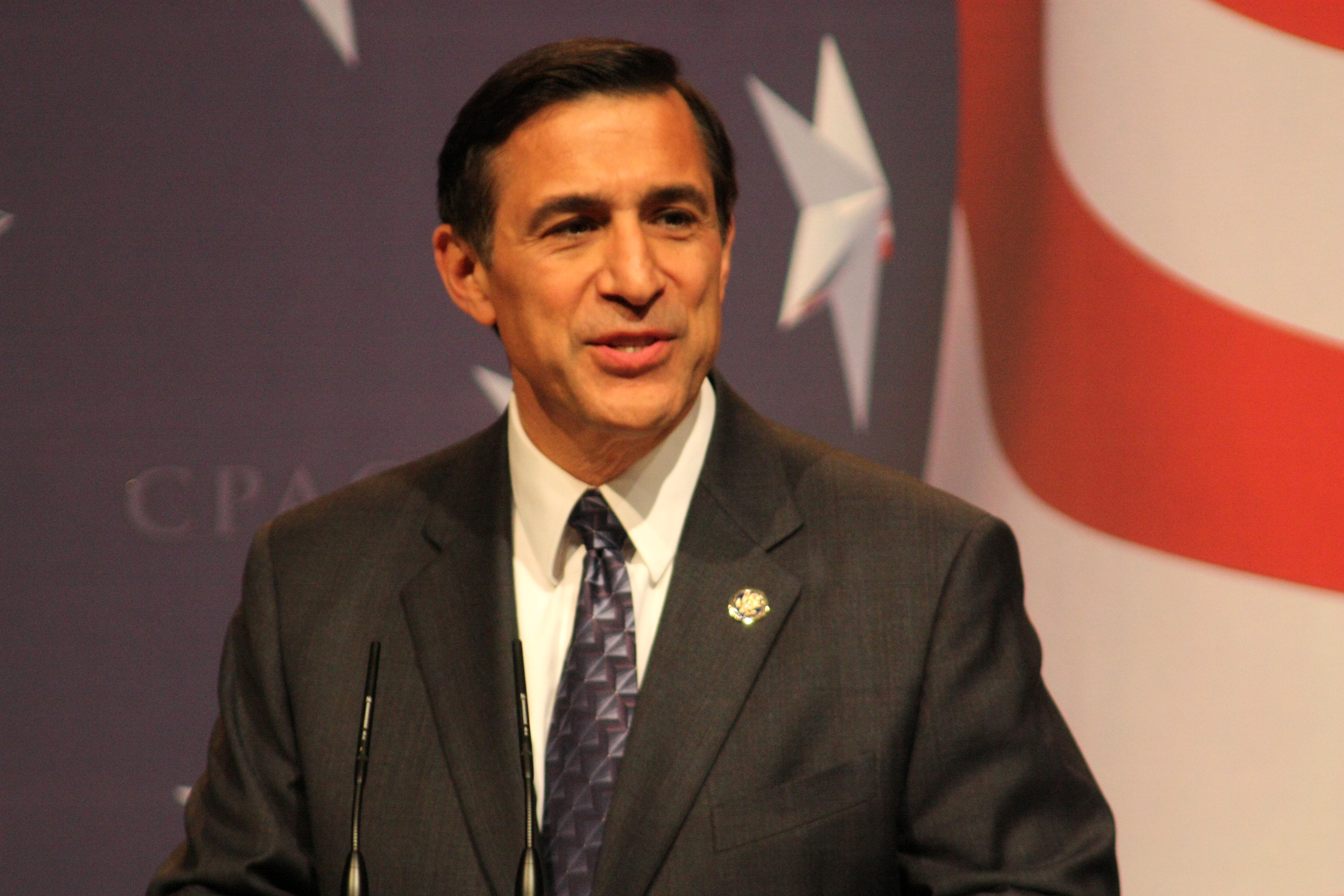This image captures Daryl Issa, a former congressman from California, standing as a speaker at a CPAC conference. He is dressed in a dark suit jacket, possibly black or dark gray, paired with a white collared shirt. His tie is a striking blue adorned with a zigzag or diamond pattern. A gold pin is visible on his left lapel. Daryl has short, dark brown hair brushed to the side, with touches of gray near his ears, and a medium brown complexion. He is looking off to the right, appearing to speak with both rows of his teeth slightly visible. In front of him, slightly to his left, are two thin black microphones. The backdrop features an American flag alongside the CPAC logo, suggesting this moment was captured during his address at the conference.